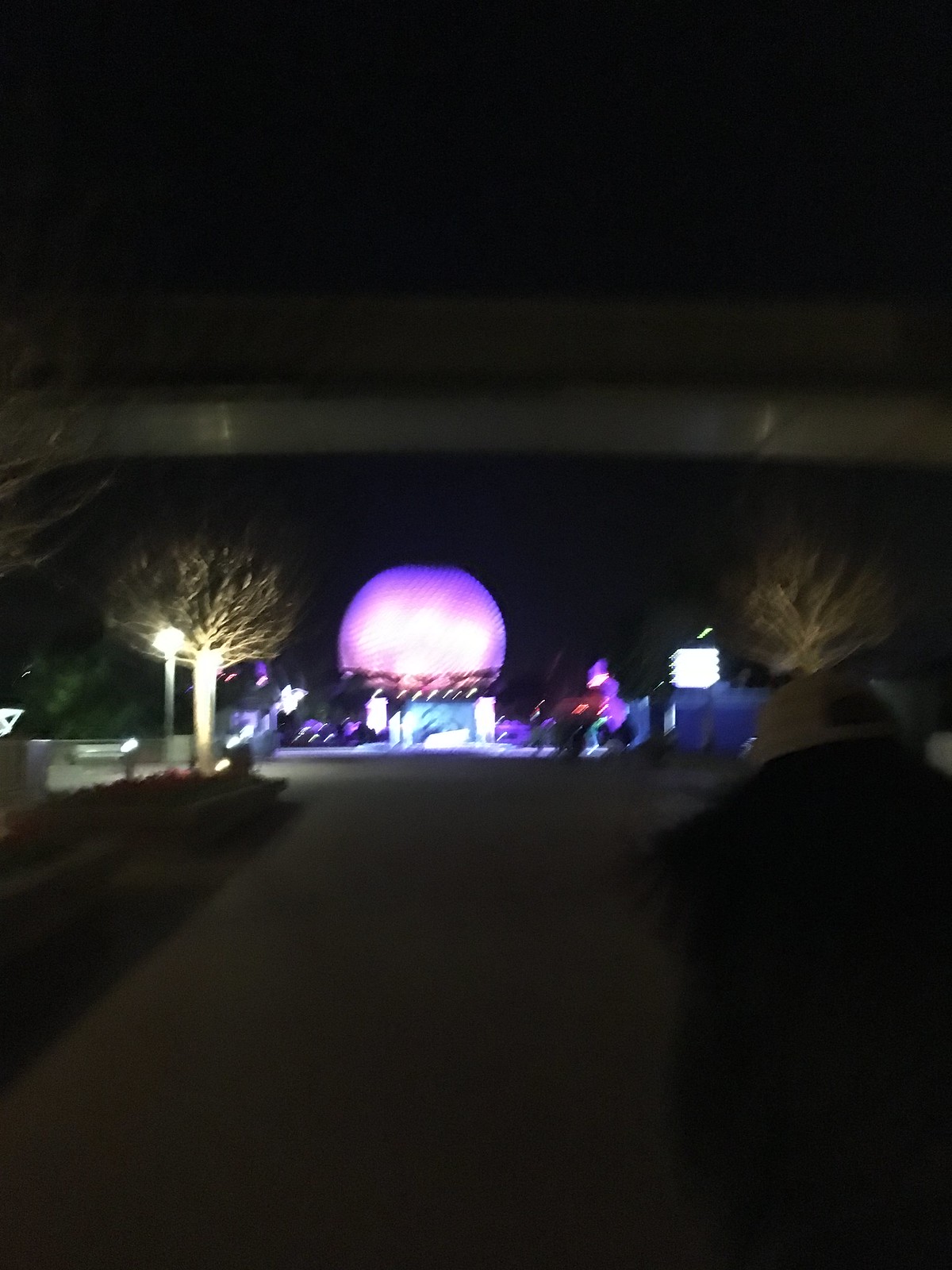In this nighttime photograph, a large, spherical structure, resembling Disney World’s Epcot Center, commands attention with its striking pink and purple neon illumination. The image, though slightly out of focus due to likely motion during capture, shows this iconic geodesic dome set against a stark black sky. The scene is framed by large trees and shadowed grass on either side of a wide concrete walkway, guiding the viewer's eye towards the lit-up entrance in the background. Elevated above the scene runs a monorail track, hinting at the park’s transportation system. To the right, a solitary person walks along the path, their presence adding a sense of scale to the grandiose structure ahead. The overall ambiance is devoid of crowds, highlighting the captivating glow of the Epcot sphere against the tranquil night.